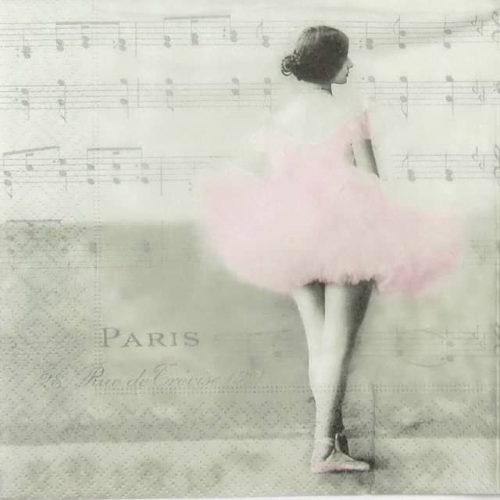This image depicts a ballerina in a graceful pose, wearing a pink tutu and matching pink ballet slippers. The ballerina is facing away, her hair neatly swept up into a bun adorned with accessories. She is slightly turned, revealing the delicate outline of her nose and mouth, but her eyes remain concealed by the soft fall of her hair. The setting is a striking contrast of monochrome and color; the overall grayscale palette of the image highlights the vivid pink of her tutu and slippers.

She appears to be transposed against a backdrop of sheet music, with at least three visible lines of musical notes behind her before they begin to fade. The sheet music creates an artistic and almost nostalgic atmosphere, suggesting a connection between music and dance. At the bottom left of the image, in the darker section under her tutu, the word "PARIS" is prominently displayed in capital letters. Below it, there are additional words—suggested to be "Rue de Arroes"—though they are blurred and difficult to decipher clearly. A subtle pattern of squares is also noted beside the text, adding to the textured and layered composition of the piece.